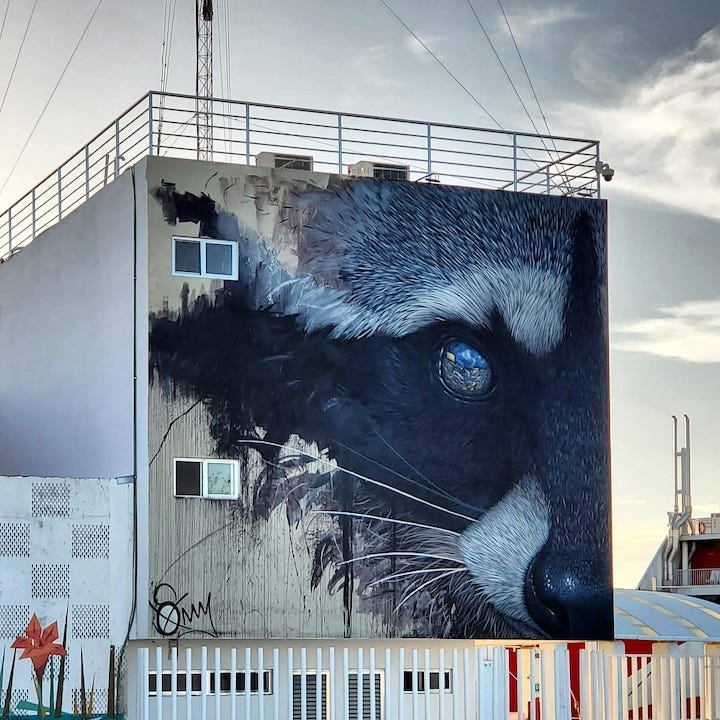The photograph depicts the side of a large, cube-shaped building with a striking mural of the right side of a raccoon's face. Taken during daytime, the image showcases a clear blue sky with a few wispy clouds. In the lower part of the image, white posts resembling a fence line the front of the building. Behind this fence, windows are visible on the ground level, while the building's upper facade is largely uninterrupted. At the top of the building, a rail runs along the roof's edge, with air conditioning or heating units visible.

The mural, located mostly on the right side of the building, is an elaborate and lifelike depiction. The raccoon's face features intricate details: a black nose, white and black cheeks, and a head that fades into gray-black smudges as it extends outward. The mural’s right eye is particularly captivating, reflecting clouds, a cityscape, and a yellowish screen. In contrast, the left side of the building has two plain windows and a possible black signature in the lower left corner. Additional interesting visual elements include the juxtaposition of lifelike details and patchy, checkerboard-like areas, contributing to the mural’s complex and arresting presence on the building.